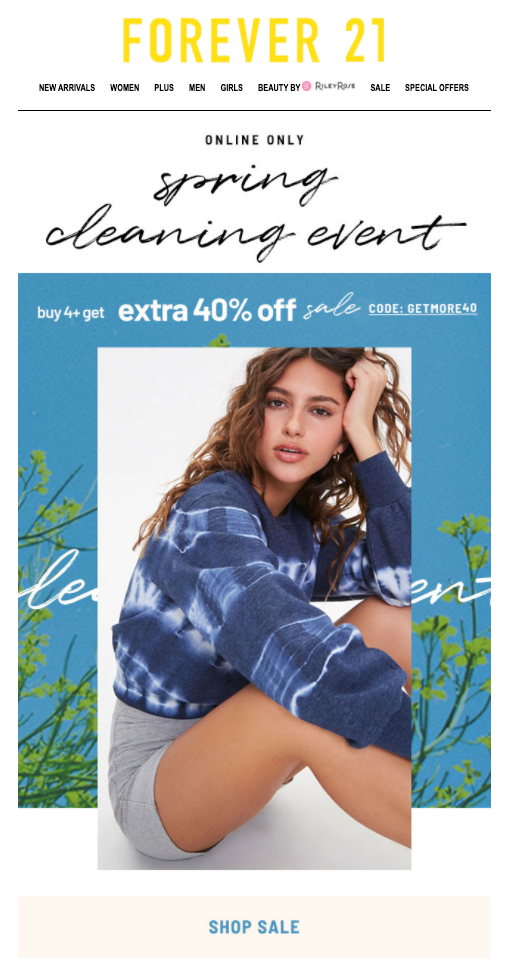The image is a screenshot of a Forever 21-like website homepage. At the top, prominently displayed on a yellow banner, is the brand name "Forever 21." Directly beneath this banner, there are navigational tabs for different sections of the website: "New Arrivals," "Women," "Plus Size," "Men," "Girls," "Beauty," "Rural Rose," "Sale," and "Special Offers." 

Below the navigation bar, there is a promotional section highlighted with the text "Online Only, Spring Cleaning Event." This promotion offers a special deal: "Buy 4+, Get Extra 40% Off Sale," accompanied by a discount code "GETMORE40." 

The main part of the page features a large image of a model. The model is sitting casually, adorned in gray shorts and a cozy blue sweater top, illustrating the stylish and relaxed clothing typical of the Forever 21 brand.